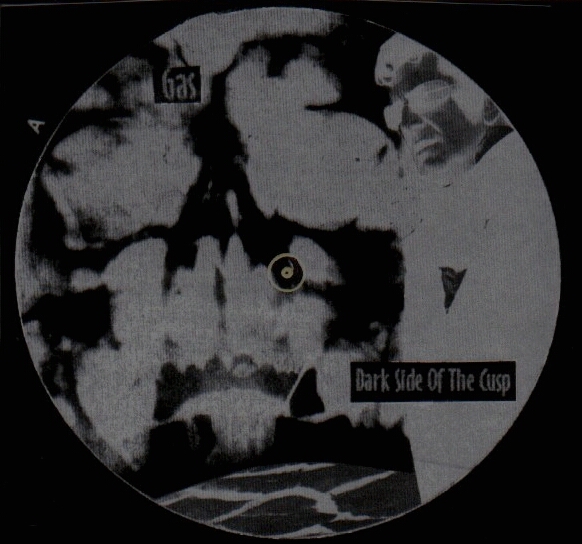The image is a digitally edited, inverted black-and-white photograph set against a completely black backdrop. In the center of the image is a circular photo resembling a zoomed-in, high-contrast negative, almost giving it the appearance of an old CD. Inside the circle, there is a man wearing sunglasses and a white shirt, sporting a curly perm. He stands on the right side, seemingly gesturing behind him. The photo has peculiar lighting effects, adding to its surreal quality.

An A symbol appears in the upper left corner of the circle. The background within the circle features what looks like an enlarged, abstract x-ray of a skull, with clouds and water faintly visible, adding layers of depth and intrigue. The flooring at the bottom has a distinct pattern. In the middle, there is a yellow dot seemingly zooming in on the man, adding a focal point.

On the upper left side of the circle, the text reads "GAS" in a white font within a black box, while on the lower right side, it says "Dark Side of the Cusp," also in white font within a black box. The overall effect is dark, muted, and highly contrasting, creating a visually compelling and enigmatic image.